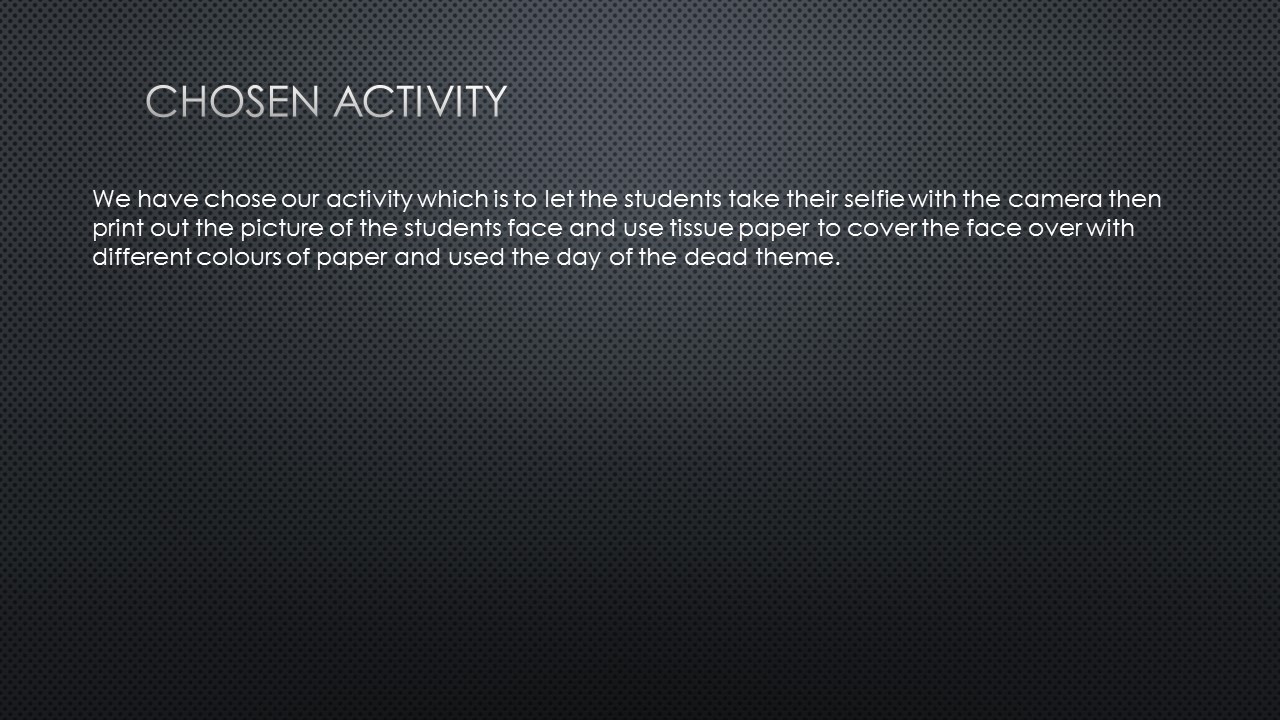The image appears to be a digital poster with a textured gray background featuring interspersed light and dark gray dots, which darken towards the bottom, creating a shiny effect in the middle. The primary text is a header positioned at the top left corner, reading "CHOSEN ACTIVITY" in all capital white letters. Below this header, a descriptive paragraph follows: "We have chosen our activity, which is to let the students take their selfie with a camera. Then print out the picture of the student's face and use tissue paper to cover the face with different colors of paper, following the Day of the Dead theme." The text maintains a professional, businesslike font and is presented entirely in white, with the heading noticeably larger than the rest of the text.